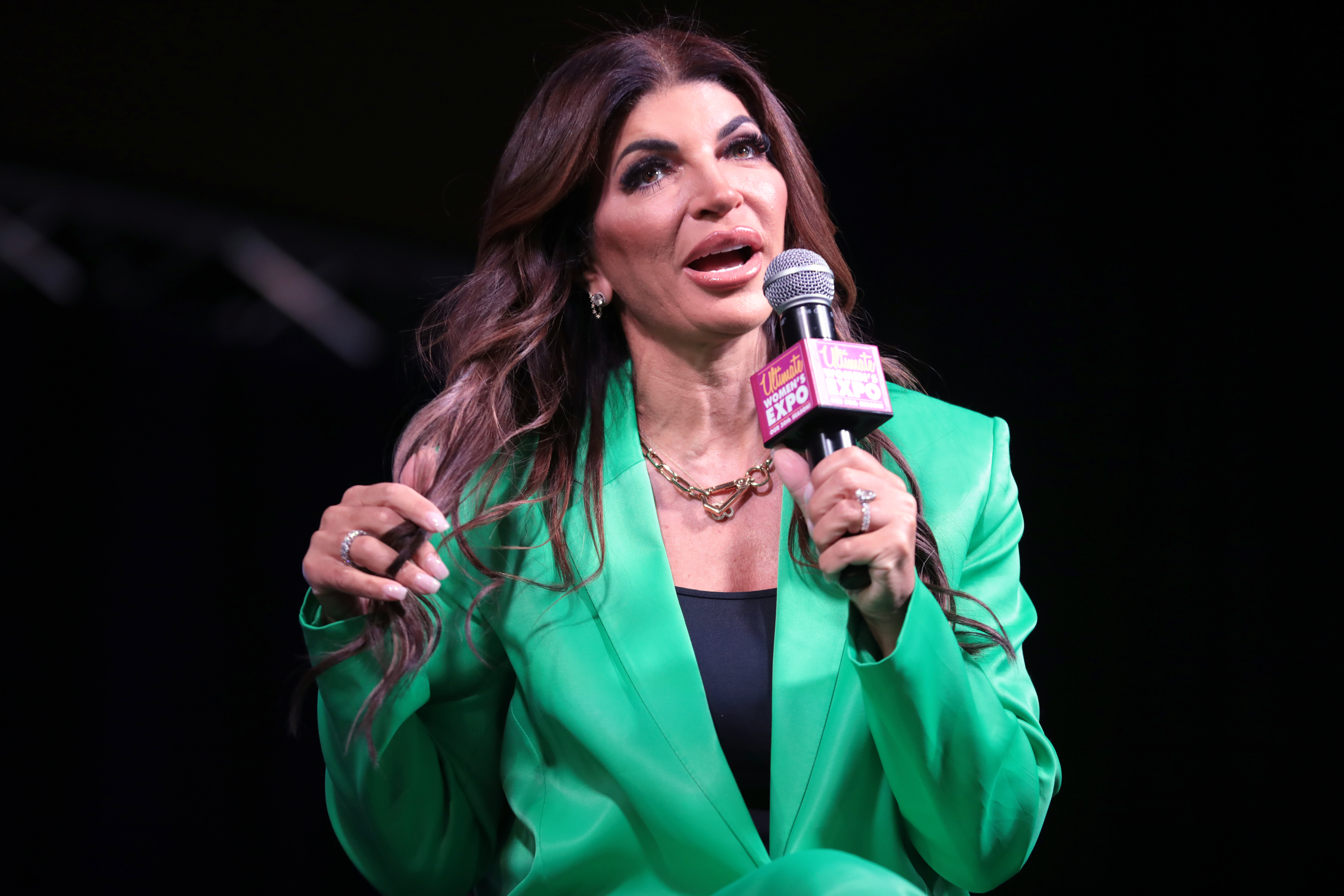The image captures a woman with long, dark brown hair who appears to be speaking at an event, as indicated by the open position of her mouth and the microphone she's holding in her left hand. The microphone, which features a pink cube with partially legible text that includes "Women's Expo," adds context to the setting. The woman is dressed in a dark blue tank top layered beneath a bright green blazer that is open in the front and buttoned around the waist. She wears a ring on her left ring finger and her right arm is bent, with her hand playfully touching her hair. Her complexion is light, and she notably appears to have had significant cosmetic work done, particularly to her lips. The backdrop is completely black, suggesting a staged environment with focused lighting, giving a clear and well-lit presentation of the subject, who is the sole person in the image.